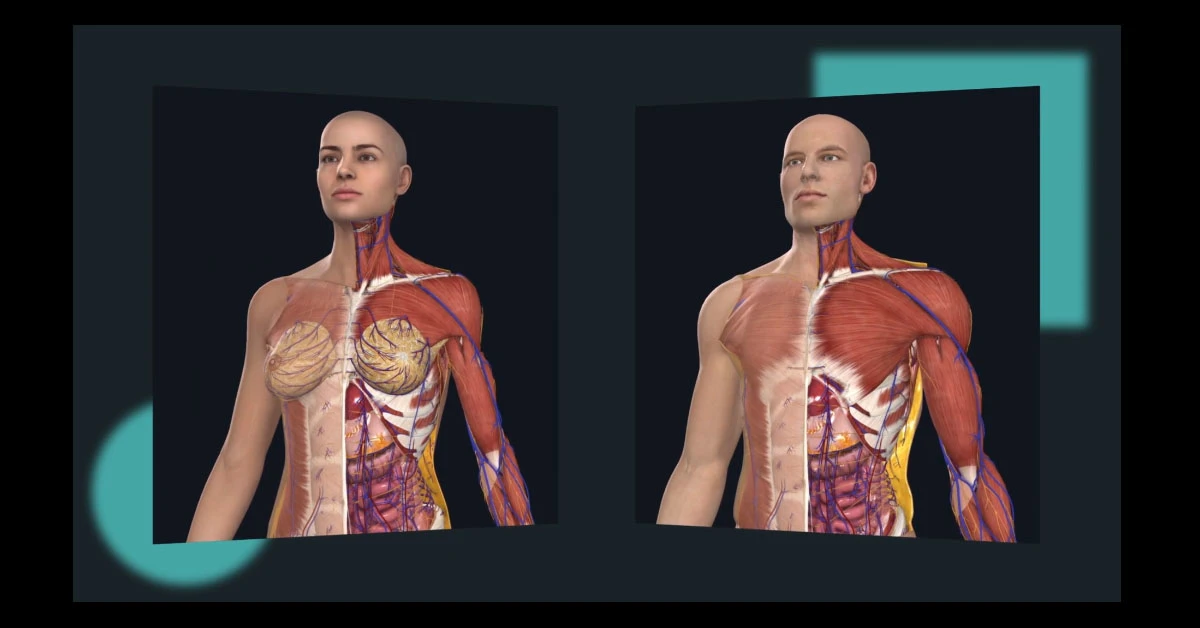This side-by-side color illustration showcases detailed anatomical renderings of a man and a woman, set against an all-black background with two squares—each featuring intricate medical imagery. The left square, encased in a dark blue background, depicts a bald man looking straight ahead, with transparent skin revealing red muscles, blue veins, and tan-colored pectoral structures. The right square displays a bald woman, similarly detailed yet slightly different, with a focus on the muscles and veins displayed in blue, but without the tan pectoral markings seen in the man's image. Both figures are presented in a realistic, AI-generated style, designed to highlight their internal anatomy, including muscles, veins, and organs, emphasizing the medical purpose of these illustrations.